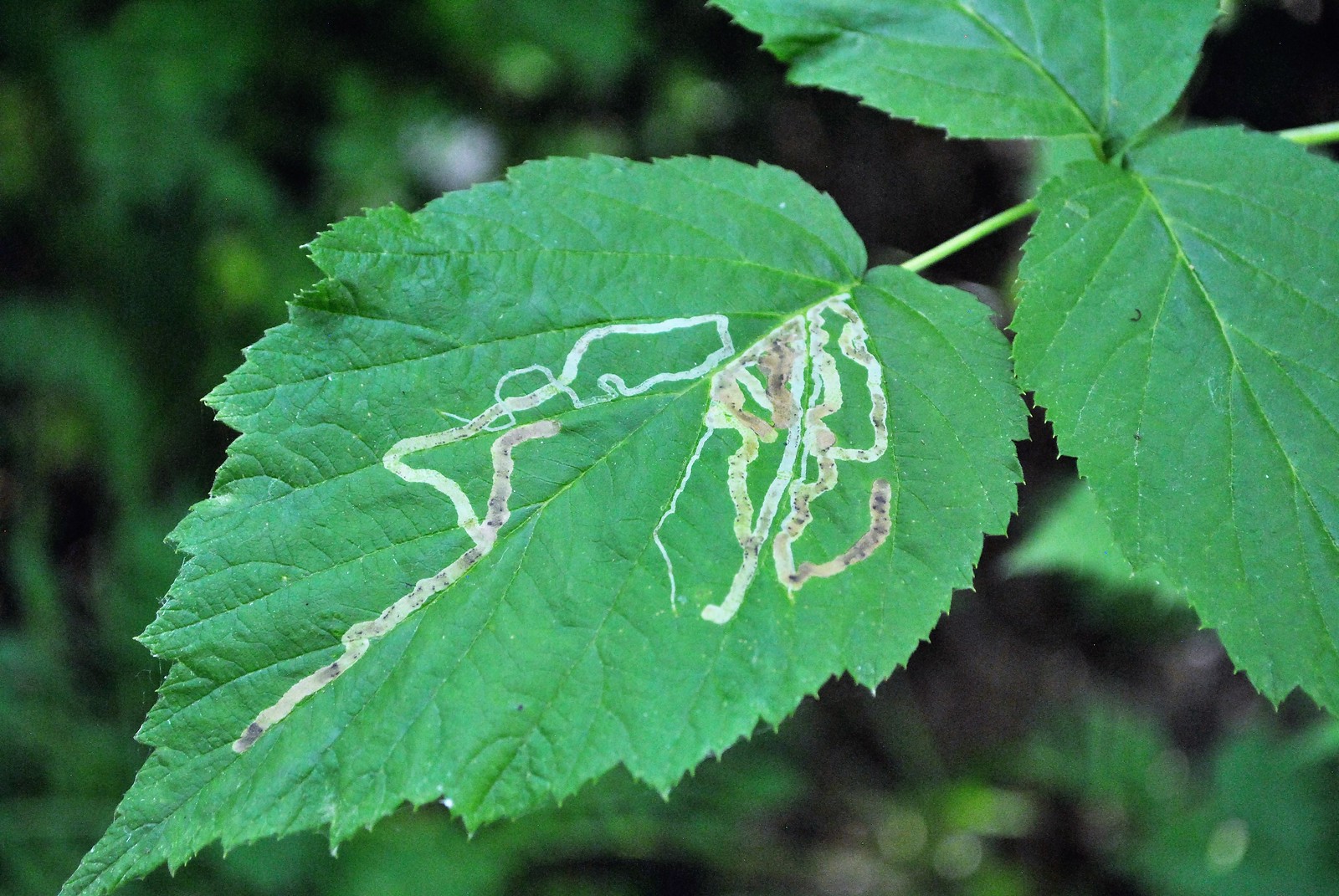This close-up daylight photograph features three prominent green leaves attached to a stem emerging from the upper right corner of the image. The composition focuses on these leaves, with the background rendered as a blurry mix of black and green hues, suggesting a wooded area but emphasizing the leaves in the foreground. The main leaf, positioned towards the lower left, displays a distinctive pattern of squiggly white or brownish-yellow lines that meander and curve across its surface. This pattern suggests the presence of a disease or damage from an insect, creating a worm-like appearance. The two other leaves extend upwards, framing the main leaf with their jagged and pointy edges. The detailed close-up captures the texture and possible afflictions of the leaves, while the blurred background draws attention to the intricate details of the plant in the foreground.